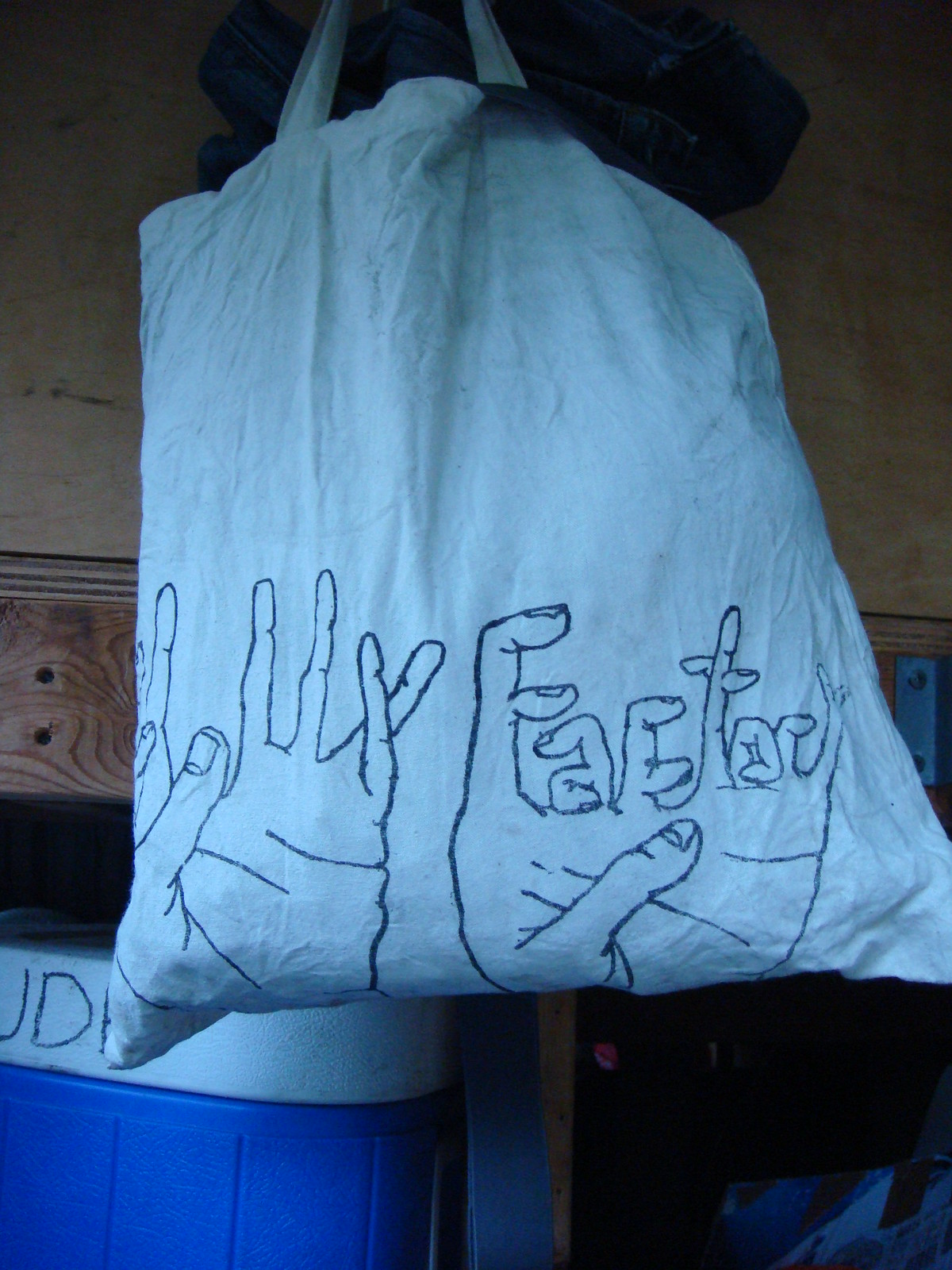This photograph showcases a white canvas tote bag, prominently displayed against a wall. The tote bag features two distinct illustrated hands at the bottom. The first hand has an unusual number of fingers, with the pinky finger and index finger crossed over each other, while the index and middle fingers form a shape resembling the letter 'U'. 

The second hand is even more peculiar, boasting about six or seven fingers curving in a manner that appears to spell out the word "factory" or potentially "Father". The overall design is eccentric and complex, making the image hard to describe in simple terms. Below the tote bag, there is a blue camping cooler with a white top, often used to store bottled water and sodas, adding a casual, outdoorsy touch to the scene. The wooden surface behind the cooler and bag enhances the rustic aesthetic of the photograph.